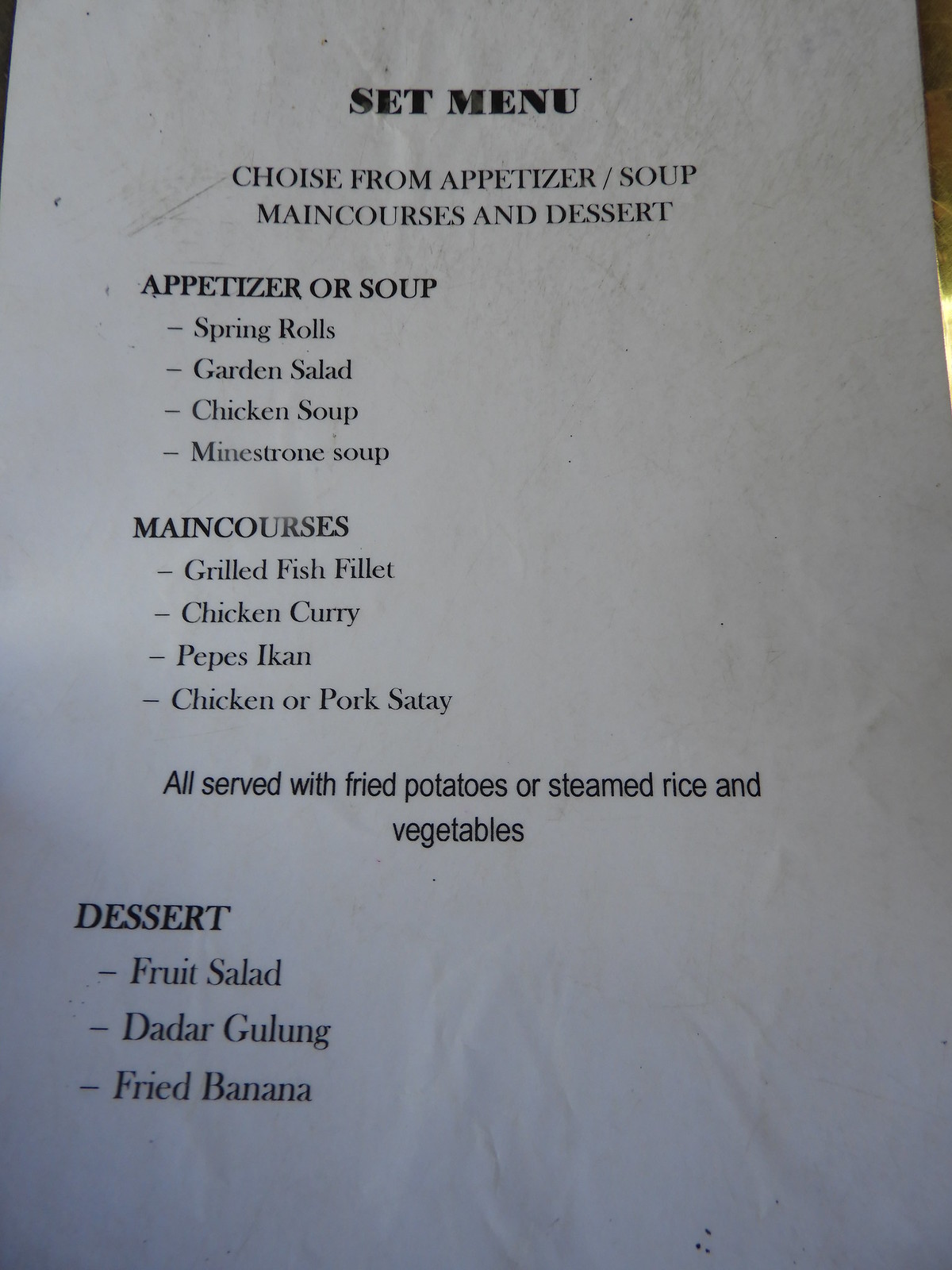In this dimly lit, quaint little restaurant, we found ourselves perusing a set menu printed on a slightly crumpled sheet of paper that might have been crafted on a typewriter. The menu, with its evident fold lines and creases, begins with "SET MENU" in bold, capitalized black text at the top. Below, it instructs diners to "CHOOSE FROM APPETIZER, SOUP, MAIN COURSES, AND DESSERT," also in all caps but not bold. The section headers, "APPETIZER OR SOUP," "MAIN COURSES," and "DESSERT," are again in bold. 

The appetizer or soup options include spring rolls, garden salad, chicken soup, and minestrone soup. For the main courses, one can choose from grilled fish fillet, chicken curry, Pepe’s Icon (a dish shrouded in mystery), and chicken or pork satay. Each main course is served with fried potatoes or steamed rice and vegetables. For dessert, the offerings are fruit salad, dadar gulang, and fried banana. The menu's eclectic array suggests influences beyond traditional American cuisine, hinting at an Indian-flavored or styled dining experience.